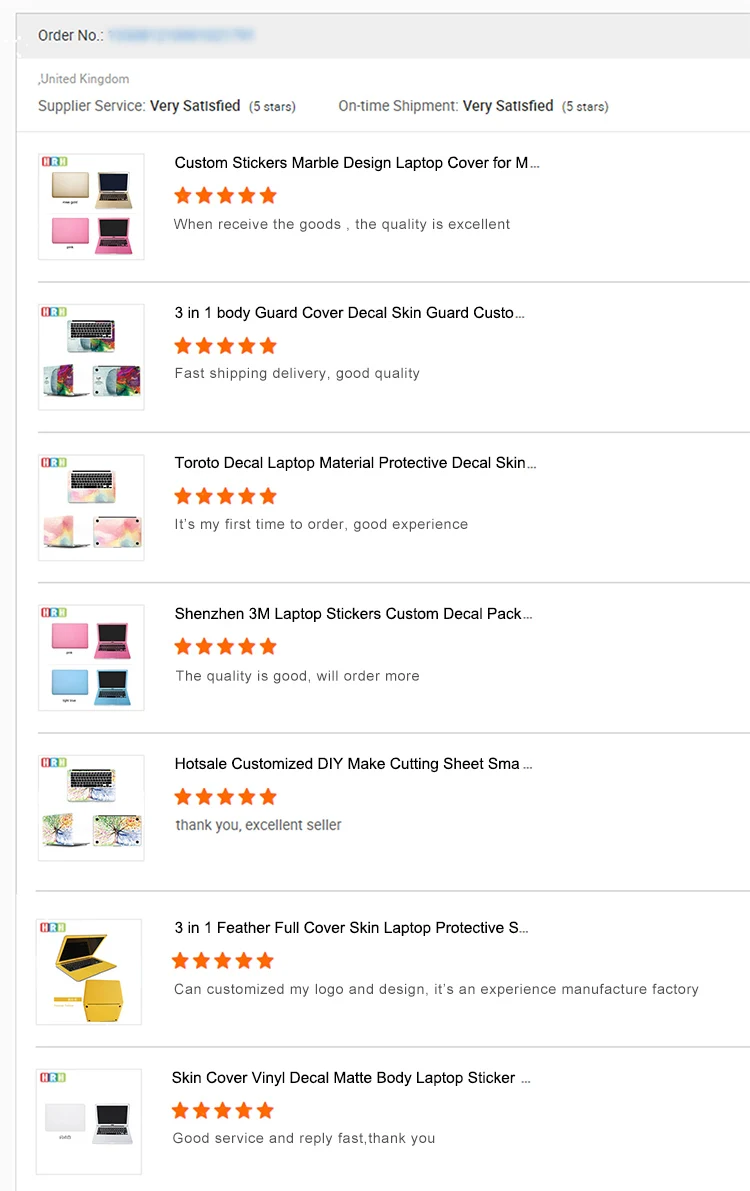The image depicts a detailed page of search results from an online order, primarily for laptop accessories, prominently featuring customer reviews. 

At the top left corner, there is an order number highlighted in blue, although it has been obscured for privacy. Directly below, the information indicates the order was placed in the United Kingdom through supplier services, receiving high satisfaction ratings—five stars for both the shipment and service.

The main content begins with a photograph showcasing multiple laptops in pink and silver colors, accompanied by the description "Custom Sticker Marble Design Laptop Cover." This entry continues with a high rating of five stars, followed by the noted remark, "Received the goods, the quality is excellent."

A dividing line separates this review from the next, which features an image of three different laptops. The accompanying description reads, "Three in One Body Guard Cover Decal Skin," and it too garners a five-star rating, praised for "fast shipping, delivery, and good quality."

Following this is another photograph illustrating three views of a laptop, linked with "TOROTO Decal Laptop Material Protective Decal Skin," earning another five-star review. The reviewer mentions, "It's my first time to order, good experience."

The final section includes four views of a laptop—two in pink and two in blue, with each color shown both open and closed. The description labels this as "SHENZHEN 3M Laptop Sticker Custom Decal Pack," which also holds a five-star rating. The review notes, "The quality is good, will order more."

Overall, the detailed reviews emphasize high satisfaction and quality across various laptop decal products.